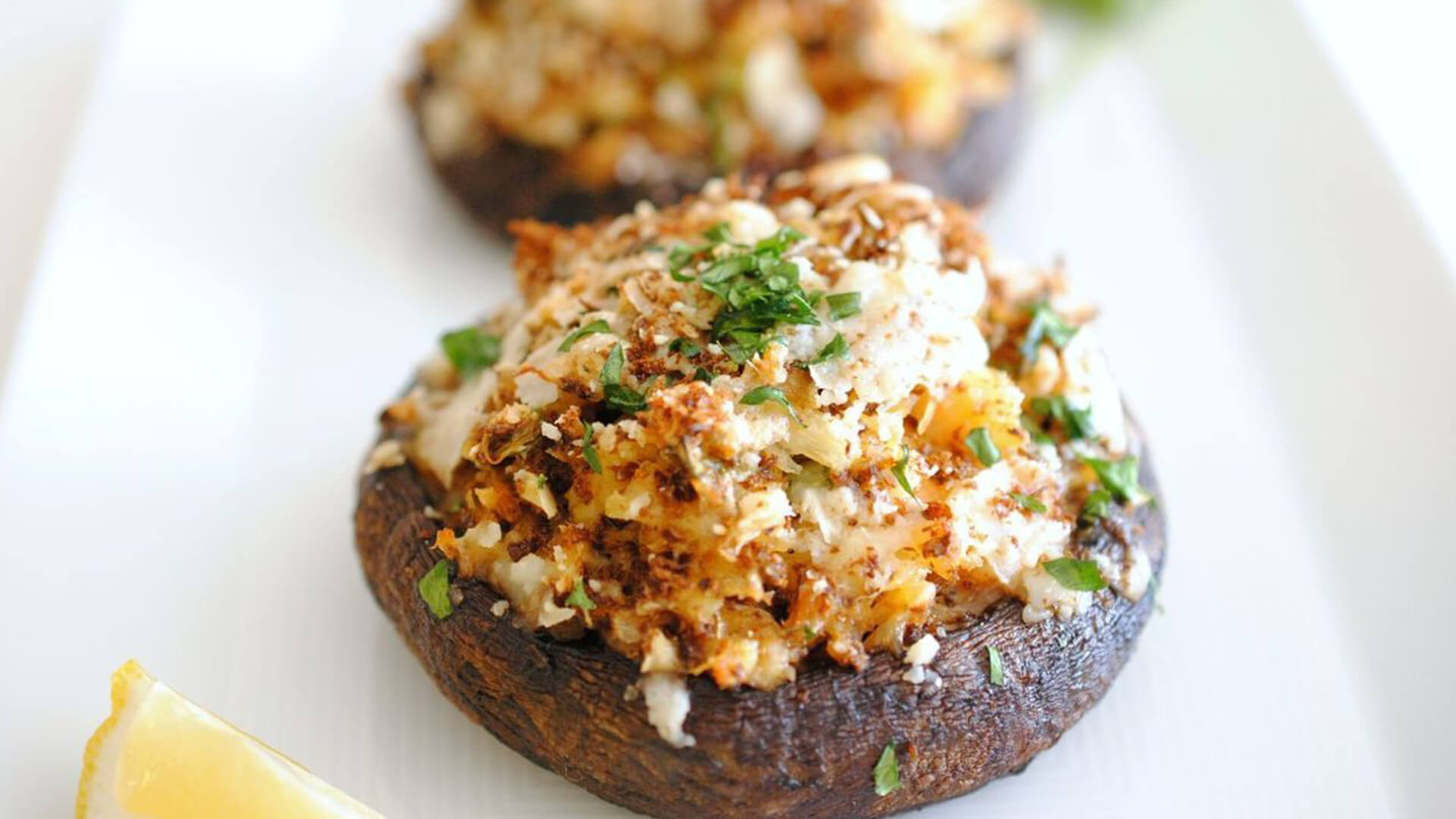This is a close-up horizontal rectangular image of a stuffed mushroom dish, positioned on a white plate against a subtly blurred white countertop background. The foreground presents a large, dark brown mushroom, centrally featured and showing off a savory filling that appears to consist of light brown breadcrumbs or crab meat, mixed with chopped green onions, parsley, and white flakes, all creating a mashed potato-like consistency. The filling is heaped generously inside the mushroom, enhancing its appetizing look. Next to the main mushroom, towards the bottom left of the image, there's a lemon wedge and a portion of a yellow napkin with a lattice pattern, adding a touch of bright color to the composition. Behind the primary mushroom, there seems to be a second mushroom, slightly blurred but mirroring the stuffed appearance of the first. The combination of textures and colors makes this dish appear delicious and inviting, despite differing opinions on the mushroom itself.